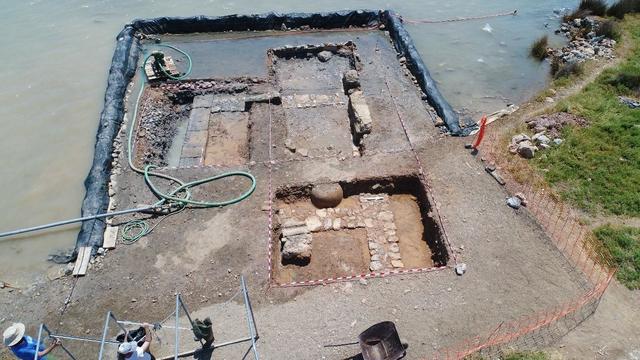An overhead aerial photograph captures an old, human-made dock situated on a murky waterway, possibly a lake. The dock features a large, squared-off area with exposed brickwork and concrete cutouts filled with stones, indicating possible demolition or drainage. A black waterproof tarp borders this area, containing the site. Several people stand near the bottom left of the image, appearing to inspect or work on the dock. An orange temporary fence is set up around the perimeter, and a pump is visible near the water's edge. The photograph also includes a patch of green grass to the right, with pathways and stones scattered around the lake's shore. A rope spans across the top of the lake, adding to the scene's complex details. The overall setting is illuminated in daylight, showcasing the intricacies of the dock and its surroundings.